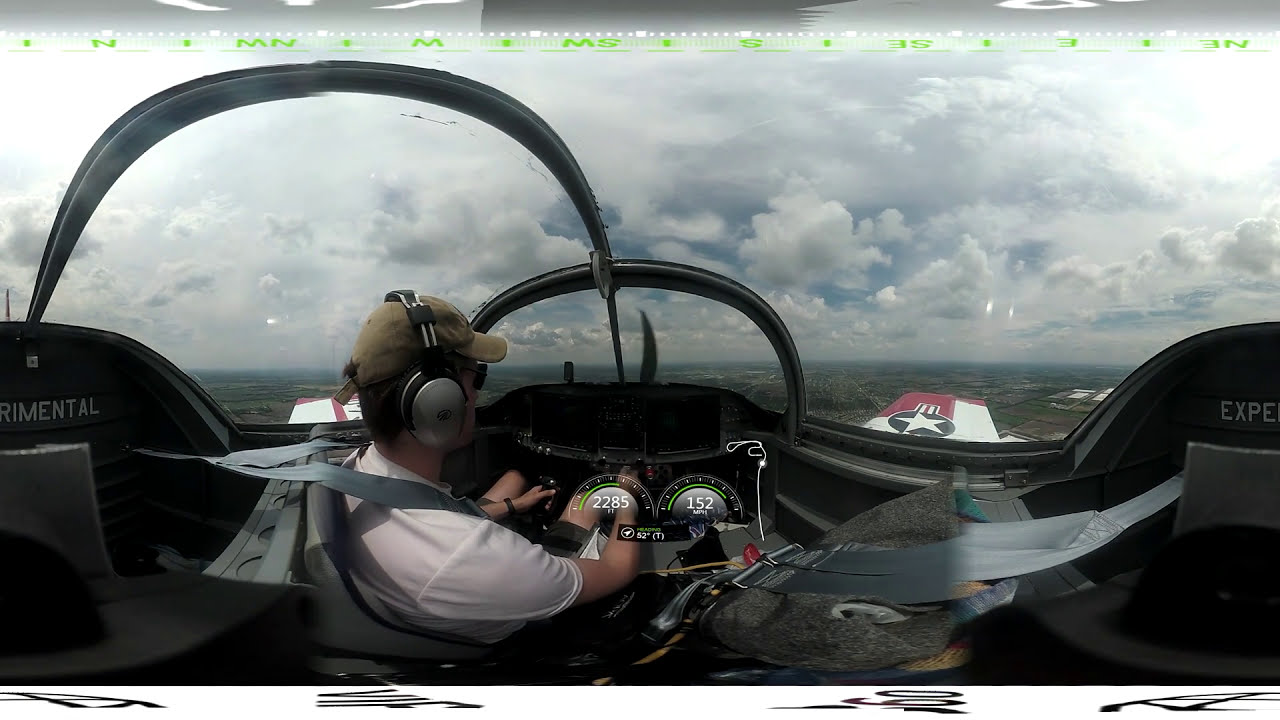The image depicts a side view inside the cockpit of a small aircraft, with a primary focus on the pilot seated centrally. The pilot is wearing a white shirt, an olive baseball cap, and headphones, and is buckled in while holding onto the controls. The cockpit features a detailed control panel in the foreground, where two dials are visible, reading 2285 and 152 respectively. To the right, the wing of the plane, colored white and red with a black circle and white star at its tip, is visible. The scene outside the cockpit showcases an aerial view of a sprawling city below and a cloudy sky above. Prominent digital banners are seen at the top and bottom of the image, emphasizing its digital nature, while no textual information is present within the frame itself. The diverse color palette includes shades of white, gray, green, red, and tan, contributing to the vibrant yet realistic rendering of a mid-flight scenario on a cloudy day.